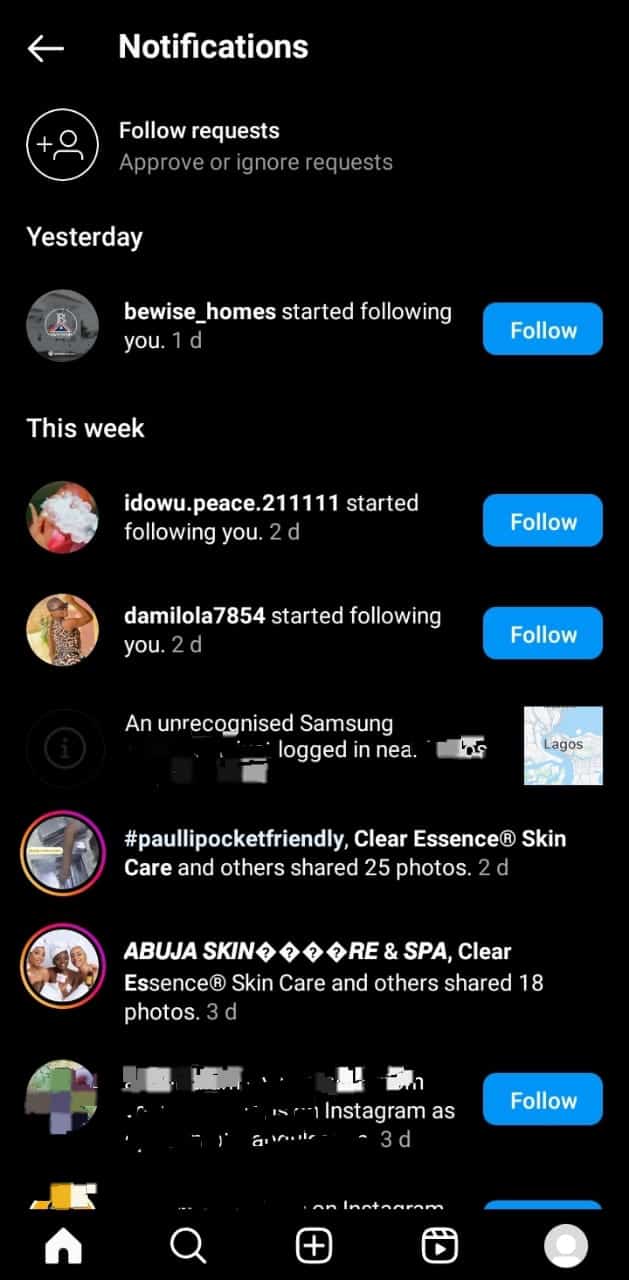**Caption:**

The image shows a series of social media notifications overlaid on a dark, pixelated background, suggesting a possible glitch. Various blue rectangular buttons read "Follow request," "Approve," "Ignore request," indicating recent follower activity. 

- "Brutalized homes started following you" (notification from yesterday)
- "This week a double P's 2 1 1 1 1 1 started following you" (notification from two days ago)
- "Down by low low 7 8 5 4 started following you" (notification with blue edges)

The text mentions "unrecognized," hinting at a potential issue or unfamiliarity with the notifications, described as "loud." It suggests that the image might have been taken with a pocket-sized device capable of sharing multiple photos, specifically mentioning locations like "Abuja" and referencing "clear essence" sharing 18 or 25 photos.

Additional icons are visible in the image: a magnifying glass, a square with a plus sign, and another square with a play button, possibly related to social media features for search, add, and video functionality.

The background is primarily black, adding to the emphasis on the glitches and icons, indicating a possible malfunction.